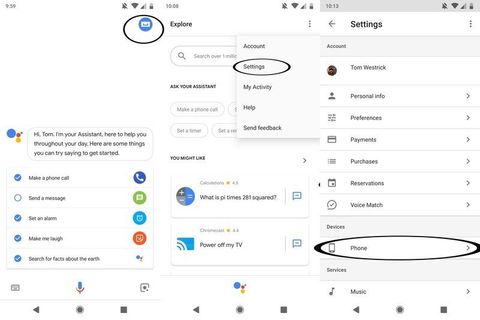The webpage features a step-by-step instructional guide with a series of three sequential screenshots from a mobile phone. Each screenshot is framed within a distinct window, creating a visual journey to assist users in navigating their device. 

In the first screenshot (leftmost window), a black circle highlights a blue icon located in the top right corner of the screen, indicating the starting point.

The second screenshot (middle window) displays a drop-down menu containing five options. A circled area emphasizes the second tab from the top, labeled "Settings".

The third screenshot (rightmost window) delves further into the Settings menu. Here, a black oval encircles the tab labeled "Phone" positioned at the bottom of the screen under the subheading "Devices", which also features a smartphone icon for easy identification.

Together, these images expertly guide users through the process of navigating to the phone settings on their mobile device.